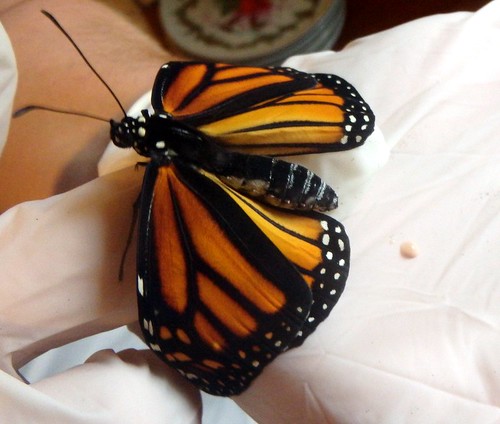The photograph showcases a strikingly beautiful butterfly, captured in reasonable detail despite not being a professional shot. The butterfly features a black body adorned with white spots, accompanied by long, black antennae. Its wings are a stunning blend of brownish-orange, brownish-yellow, and gold shades, intricately outlined in black. The outer parts of the wings are marked by distinctive black bands decorated with white polka dots, and near the tail, there are additional white stripes. The butterfly is positioned on what appears to be a white-gloved hand, potentially the tip of someone’s finger, facing left. The background is blurred and indistinct, showing a mix of red, green, white, and pink hues, but not providing any clear environmental context. The image likely captures an interaction with the butterfly in a close-up, intimate moment, highlighting its vibrant details against a soft, undefined backdrop.